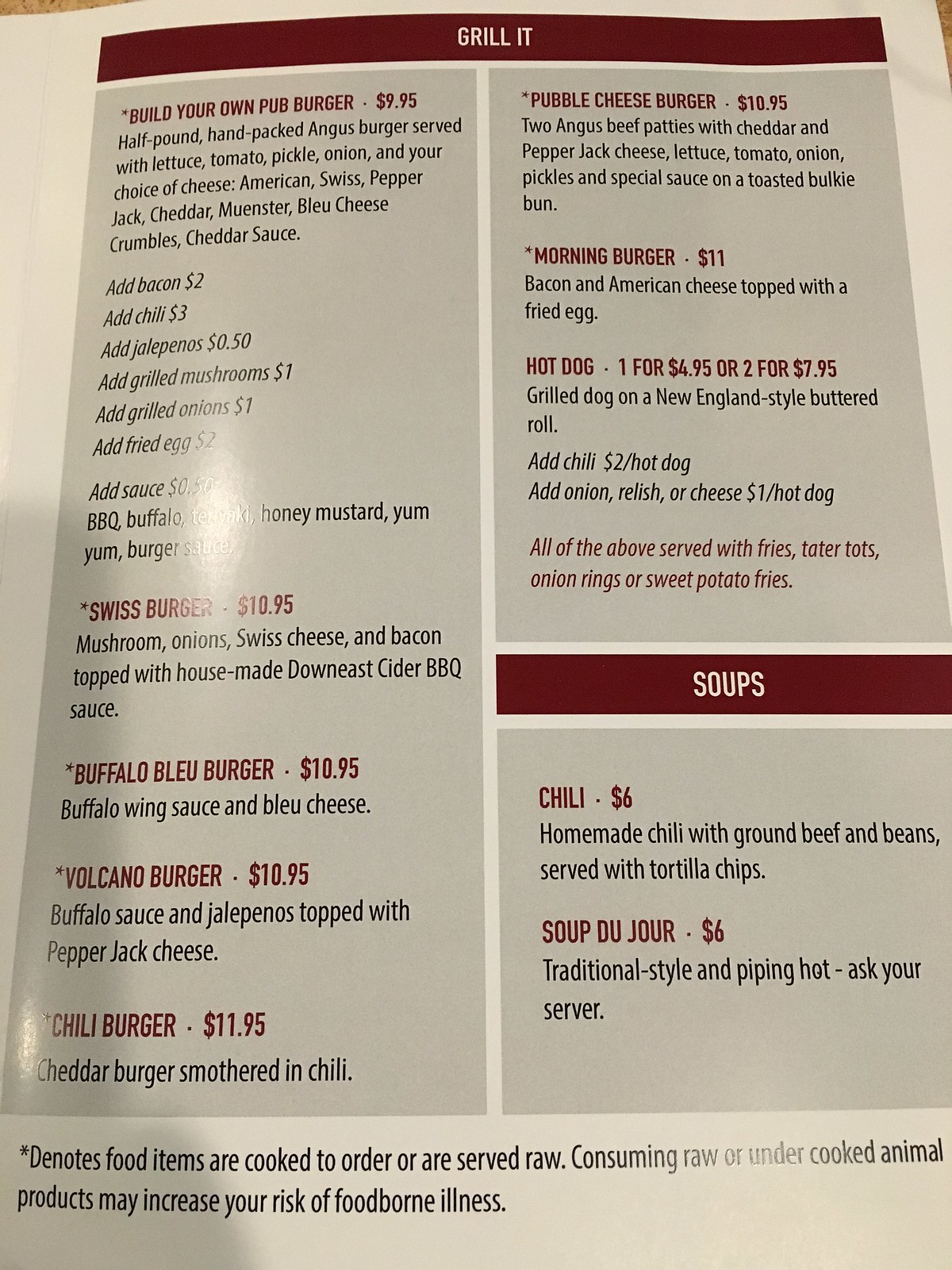**Restaurant Menu Overview – The Grill Section**

On this page of the menu, we present the tantalizing selection available in the grill section.

*Top Left*:
- **Build Your Own Pub Burger** – $9.95
  - A generous half-pound, hand-packed Angus burger served with crisp lettuce, juicy tomato, crunchy pickle, fresh onion, and your choice of cheese: American, Swiss, pepper jack, cheddar, Monterey Jack, blue cheese crumbles, or cheddar sauce. Additionally, there are various other toppings available to customize your burger to your preference.

*Base Burgers*:
- **Swiss Burger** – $10.95
- **Buffalo Blue Burger**
- **Volcano Burger**
- **Chili Burger**

*Top Right*:
- **Pubble Cheese Burger**:
  - An impressive creation featuring two Angus beef patties adorned with cheddar and pepper jack cheeses, enhanced by a special signature sauce.
- **Morning Burger**:
  - A hearty option topped with crispy bacon and a perfectly cooked egg.

All burgers are served with a choice of fries, tater tots, onion rings, or sweet potato fries, providing options to suit every taste.

*Underneath the Burgers*:
- **Soups Section**:
  - The section header "Soups" is prominently displayed in a red bar with white borders above and below.
  - Available soups include the restaurant's hearty chili and the soup du jour, which changes daily.

*Important Note*:
- An asterisk at the bottom of the menu indicates that some food items are cooked to order or are served raw. Consuming raw or undercooked animal products may increase your risk of foodborne illness.

*Design*:
- The menu features a sophisticated grayish background with a distinct white stripe running vertically down the middle, creating a clear division between the left side, showcasing various burger options, and the right side, which includes additional burger choices and the soups section.

This concise and visually appealing menu page provides all the details you need to make an informed and delicious choice at this restaurant.